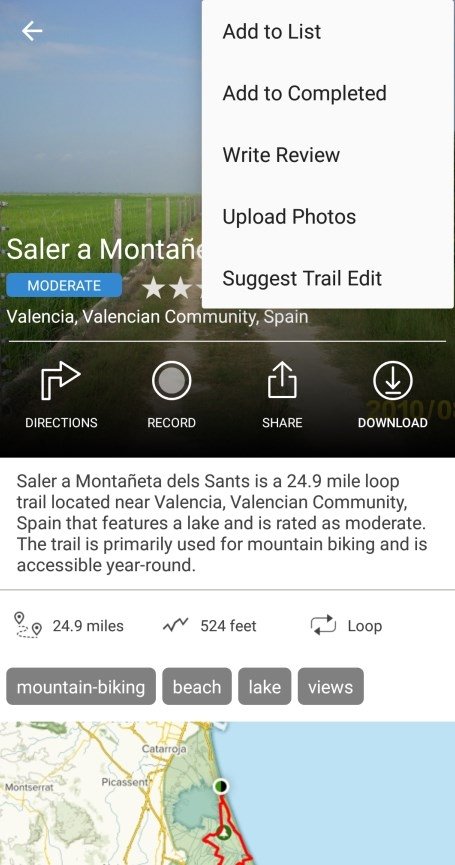This is a detailed screenshot of a webpage from an unknown site, featuring a scenic trail in Valencia, Spain. The background image showcases a serene dirt road flanked by vibrant green grass and a rustic wooden and chicken wire fence on the left-hand side. However, a drop-down window partially obscures much of the photograph and the text. The drop-down menu contains several options: "Add to List," "Add to Completed," "Write Review," "Upload Photos," and "Suggest Trail Edit."

Despite the obstruction, you can discern additional details on the screen. The overlay partly blocks a textual description and a star rating. Visible text reads: “Valencia, Valencia Community, Spain,” with accompanying icons for "Directions" (indicated by a right-facing arrow), "Record" (symbolized by a circle), "Share," "Upload" (a white box with an upward-pointing arrow), and "Download" (a white circle with a downward-pointing arrow over a horizontal line).

The primary focus of the screenshot is the description of the “Salar a Montañeta del Sanz” trail, a 24.9-mile loop located near Valencia. It features a lake and is rated as a moderate trail, mainly used for mountain biking, and is accessible throughout the year. Key trail attributes include: 24.9 miles in length, an elevation gain of 524 feet, and it offers diverse landscapes like beaches, lakes, and panoramic views. There is a partially visible map at the bottom of the image, hinting at the trail's layout and starting point.